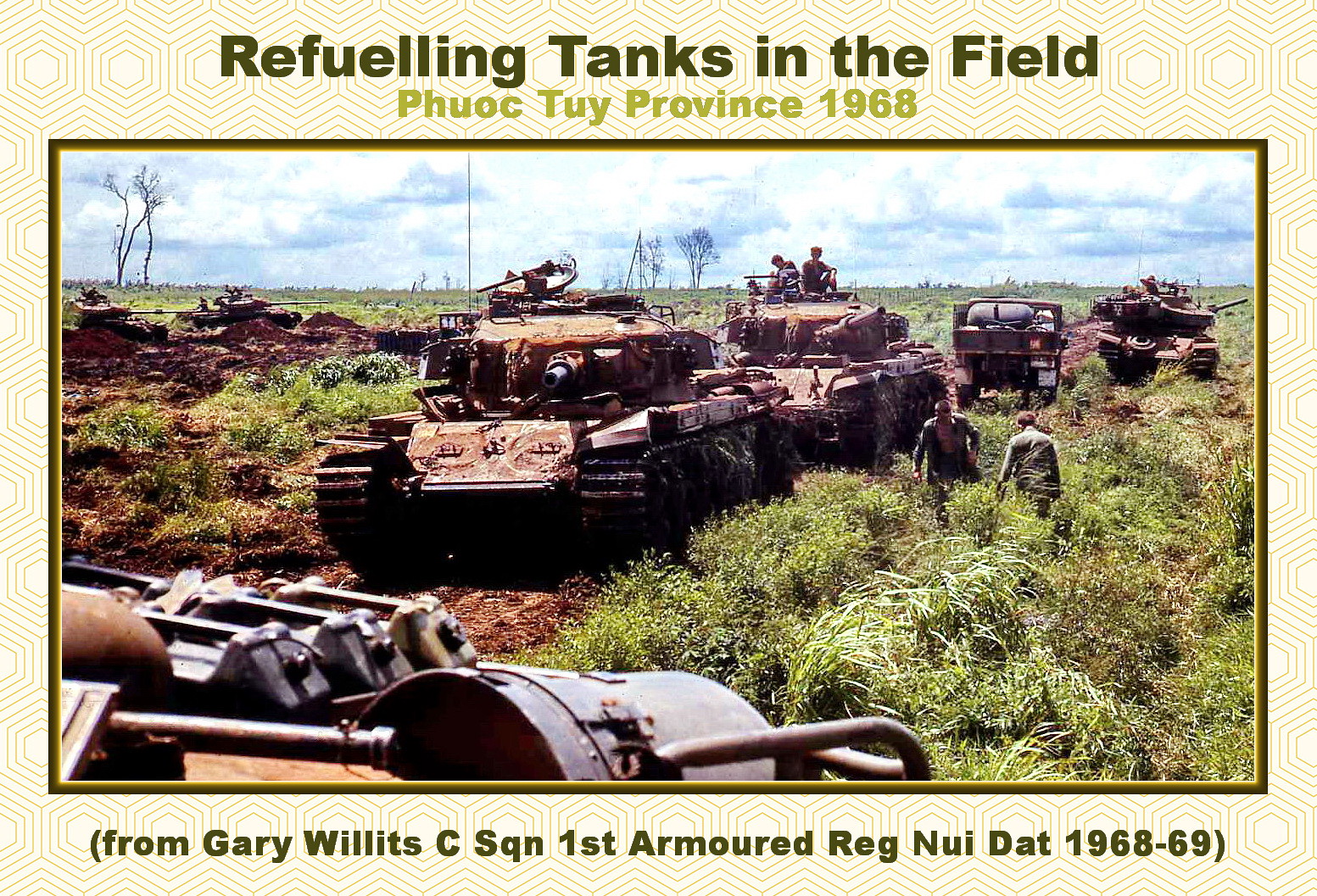This full-color photograph, taken during the Vietnam War in 1968, depicts a scene in the daytime in Phuoc Thuy Province. The image captures several army tanks positioned in a muddy, grassy field, visibly torn up by their tracks. In the foreground, a tan, brown, and gray tank is prominently displayed, while two more tanks follow behind, and another vehicle, possibly a truck, is partially visible. On one of the tanks, two men are seated, and in the background, two more men stand in the grass. Tall green grass interspersed with patches of brown mud and some dead trees in the far distance paint a stark contrast against a bright light blue sky adorned with fluffy white clouds. The top of the photograph is labeled in green text, "Refueling Tanks in the Field, Phuoc Thuy Province, 1968," and at the bottom, it reads, "From Gary Willett's C-Squadron, 1st Armored Regiment, July 1968 to 1969."